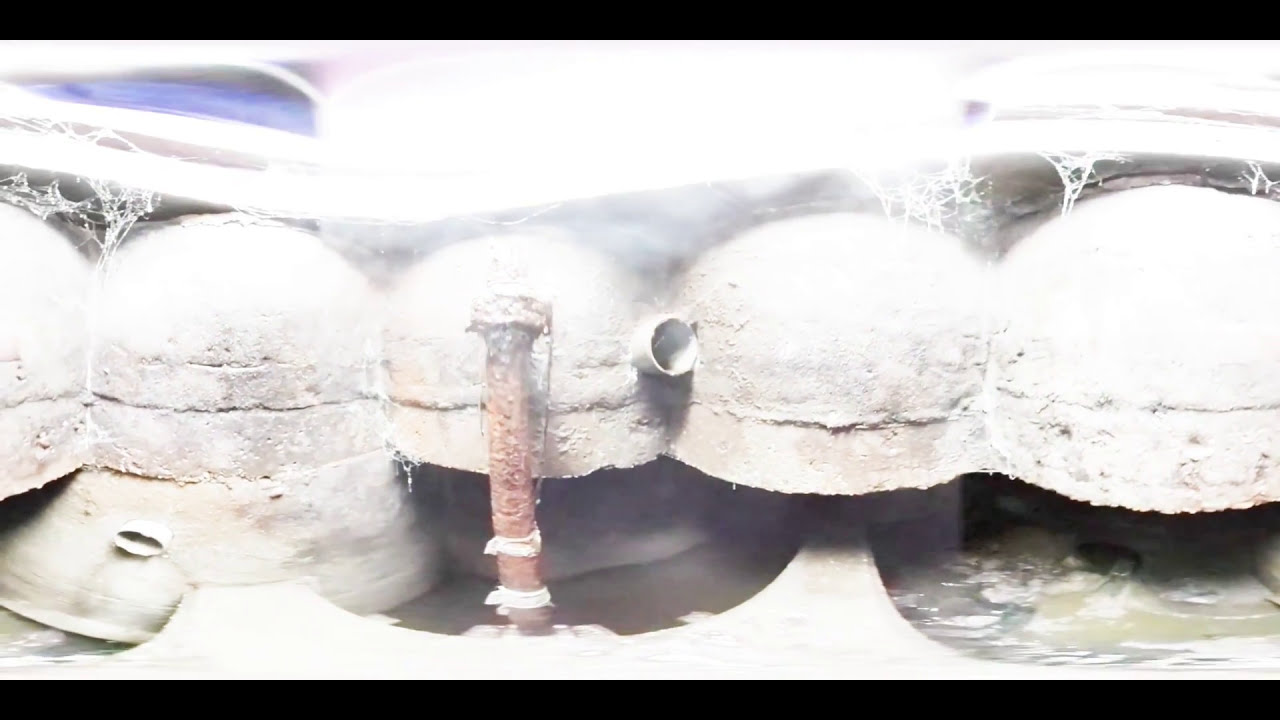The image depicts five white, bell-shaped structures that resemble upside-down cups or old flapper hats from the 1920s and 30s. These structures, which may be made of clay, rock, concrete, or stone, are lined up in a slightly cave-like setting. A notable feature in this scene is a reddish-pink object, identifiable as an old candlestick, leaning against the third structure. Additionally, a rusty iron bar or spike rests in front of one of the middle structures, contributing to the aged and abandoned ambiance. The scene is draped with numerous cobwebs, suggesting it has been left untouched for some time. The photo appears to be captured with a mobile device and is wider than it is tall, framed by thin black bars at the top and bottom. The lighting is quite bright at the top of the image, with a few lines visible on both sides. The overall impression is one of decay and neglect, adding a mysterious, historical atmosphere to the photo.